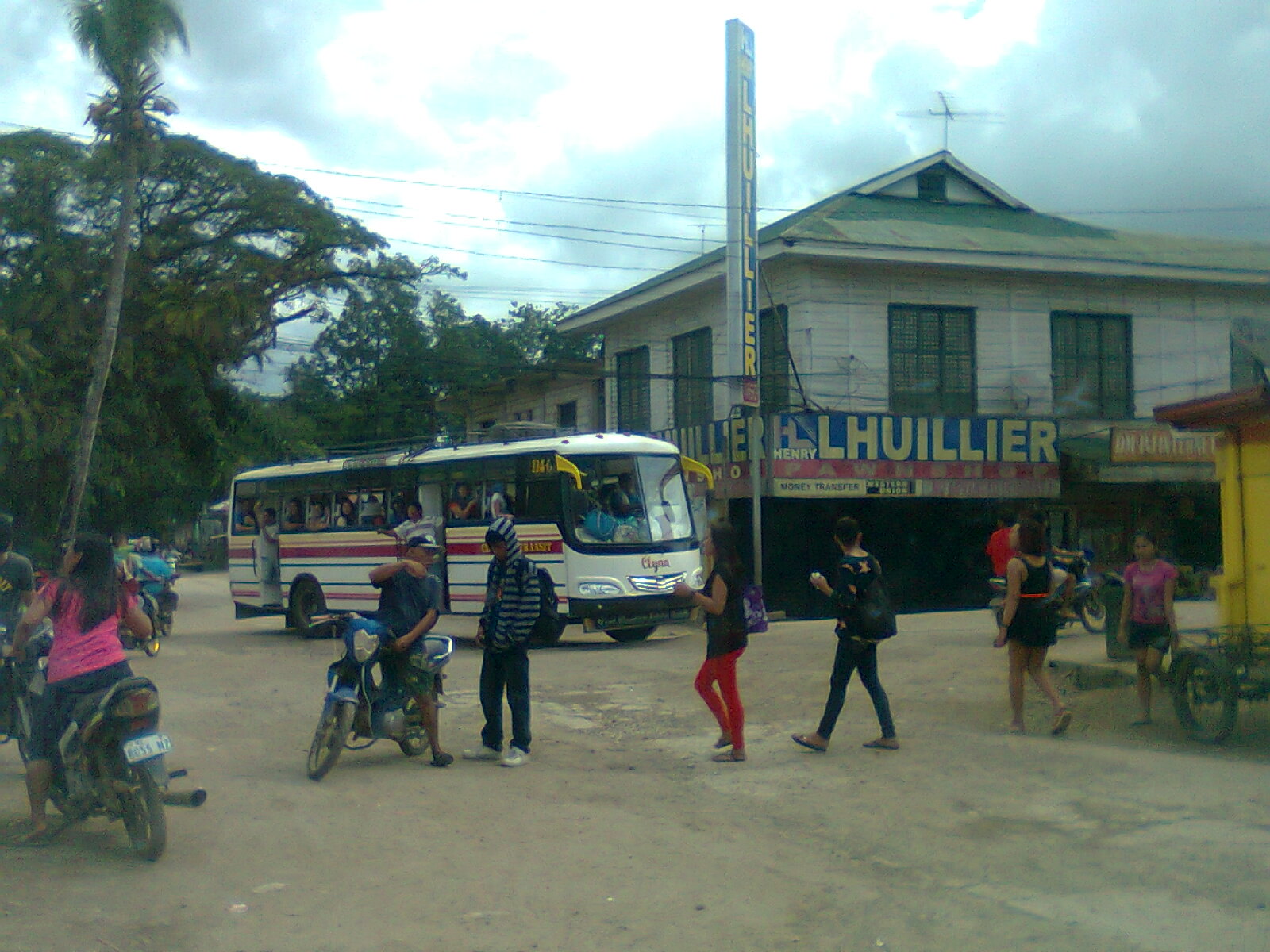In this urban scene, likely set in Mexico or South America based on architectural and environmental cues, a busy street unfolds against a backdrop of a slightly rundown building. The building, painted off-white with a green roof and green shutters, displays multiple signs: a blue and yellow banner that reads "H-U-I-L-L-I-E-R," a red “Pawn Shop” banner, and a yellow “Money Transfer” banner with a Western Union logo. The street, composed of dirt, sets the stage for a bustling intersection under a mostly overcast sky with occasional sunlight peeking through, indicating an impending rain. 

A large white city bus adorned with horizontal stripes of yellow, red, and blue is seen turning a corner. Around the bus, seven individuals mill about, two of whom are riding small bikes or mopeds, while the remainder walk in simpler attire. On the left, trees add a touch of greenery to the otherwise gritty urban landscape, and on the right, a glimpse of a yellow structure peeks through. The overall scene suggests a lively, modestly resourced community engaging in their daily routines amid the slightly gloomy weather.